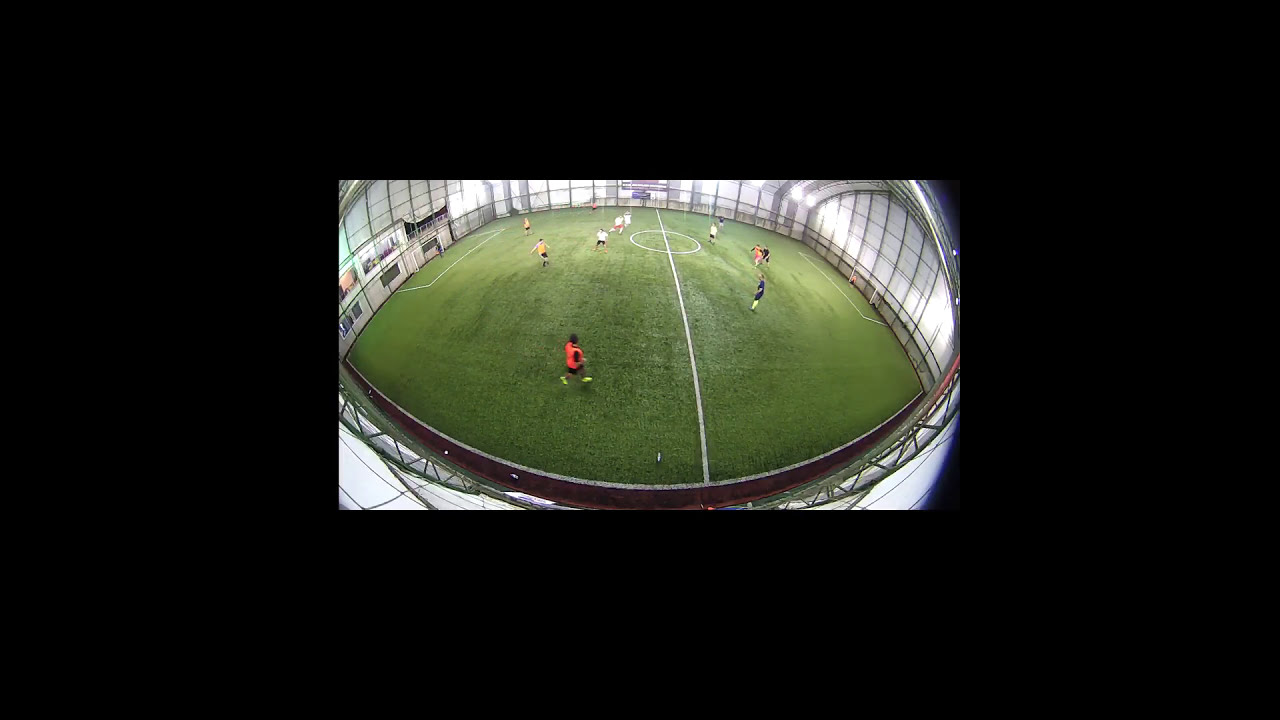The image depicts a small-resolution, wide-angle, fisheye view of an indoor soccer pitch, enclosed in a dome-like structure. The photograph is framed by a black border and appears to be captured from webcam footage. The green field, likely AstroTurf, features a white line down the center and two goals at either end. The structure is supported by steel columns, ensuring the dome maintains its shape. On the field, there are eight players dispersed, likely in a four-on-four match. The players are wearing white, yellow, and orange pennies, making them somewhat distinguishable despite the small size and distance of the image. The arena resembles a large indoor hangar with white walls and multiple windows at field level, possibly for coaches or instructors to observe the game. Spectator seating is absent, emphasizing the venue's focus on the game itself.